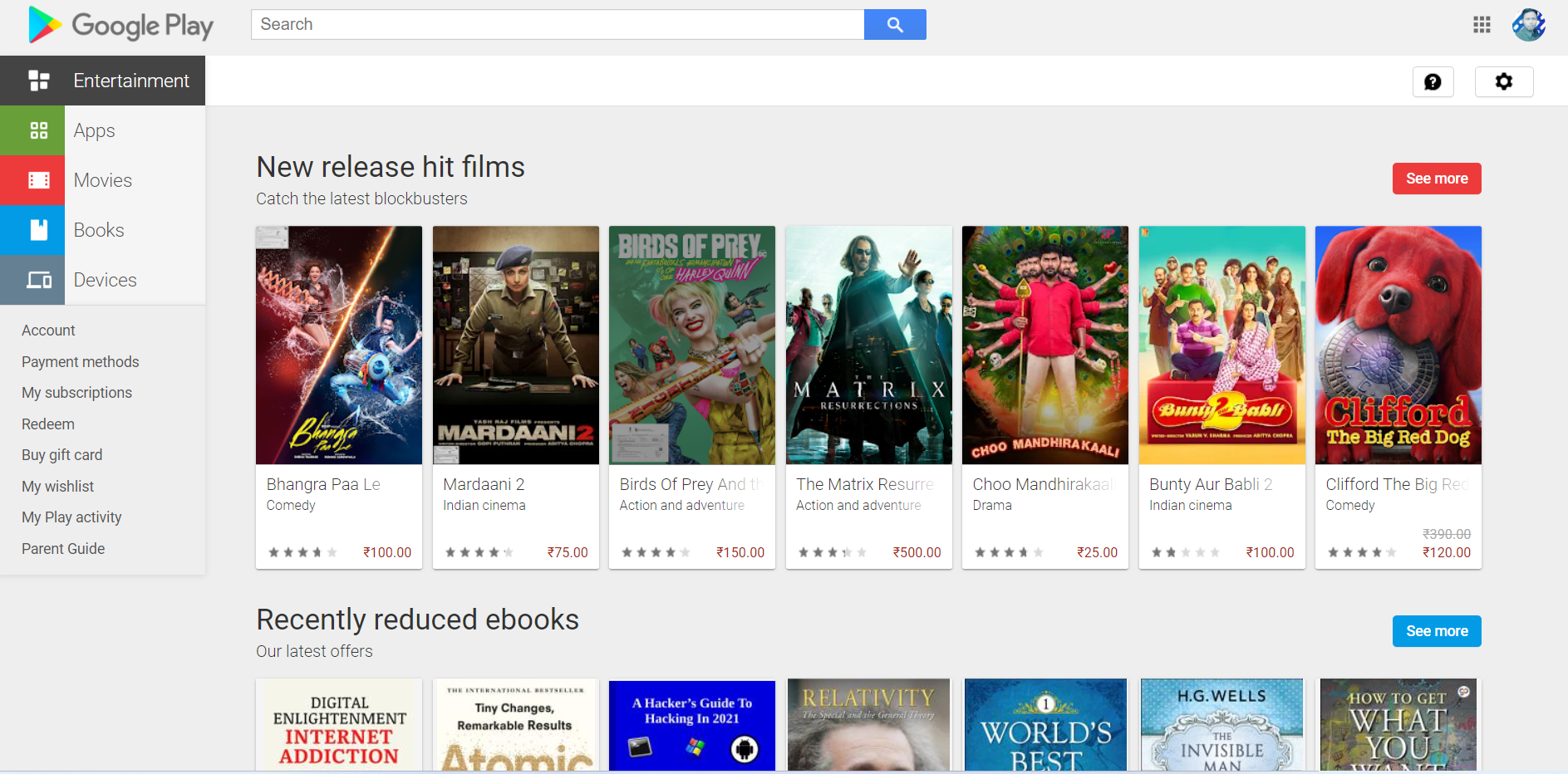In the top left corner of the image, there is a stylized arrow composed of blue, red, and yellow colors. To its right, the text "Google Play" is displayed in bold black letters. Adjacent to this, there is a long search bar accompanied by a blue square icon.

Beneath these elements, a headline reads, "New Release Hit Films," inviting users to "Catch the latest blockbusters." Below this text, several movie thumbnails are presented in a horizontal array.

The first square showcases an action movie poster featuring a character riding a futuristic blue vehicle, seemingly traversing through space. The next thumbnail is for the movie "Mardaani 2." Adjacent to it, there is a poster for "Birds of Prey," starring Harley Quinn. Following this is "The Matrix Reloaded," with Keanu Reeves in his iconic role wearing a long black coat and extending his hand outward.

To the right of "The Matrix Reloaded," there is another film titled "Chew Drama." The next movie is "Bunty Aur Babli," and finally, on the far right, there is an image of "Clifford the Big Red Dog," featuring the titular character with bright red ears, a black nose, black eyes, and a Frisbee in his mouth.

On the left side of the image, there is a vertical block labeled "Entertainment." Beneath this, there are categories listed: apps, movies, books, and devices.